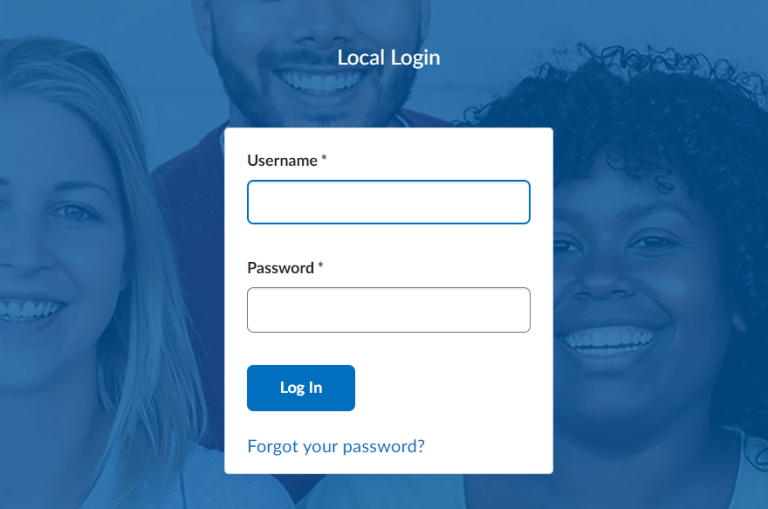The image is a screenshot of a login page on a website or application. The background features a photograph of three individuals, though their faces are partially cut off. From left to right, there is a blonde white woman whose face is partially visible, showing her left side and shoulder. Next is a light-skinned man with a beard, depicted with his face cut off just above the nose. To his right is a smiling black woman with curly hair, whose face is mostly visible except where it is obscured by the login window.

The entire background image has a blue filter, giving it a uniform blue tone. The login box itself has a white background. At the top of the login box, "Local Login" is written in white text. Inside the box, there are two input fields: the first labeled "Username*" with a blue-outlined text field below it and the second labeled "Password*" with a light gray-outlined text field beneath. At the bottom of the login box, there is a blue "Login" button with the word "Login" in white text. Below this button, "Forgot your password?" is written in blue text.